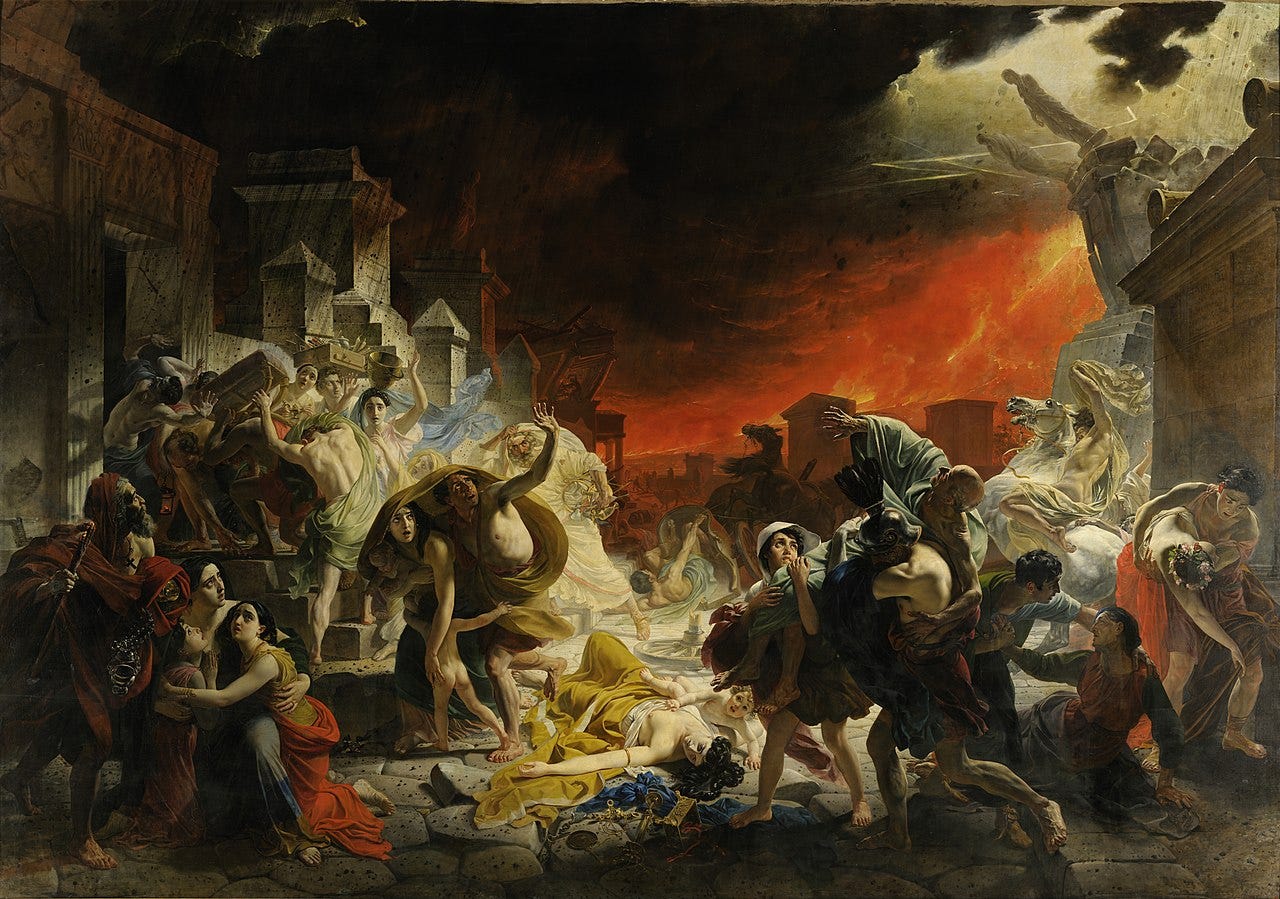This is a detailed painting capturing the dramatic moment when Pompeii was engulfed by the eruption of Mount Vesuvius. The ancient Roman city is depicted outdoors, filled with people in terror, fleeing from the imminent destruction. Amid the chaos, buildings crumble and statues fall, overwhelmed by the flowing orange lava and billowing smoke from the volcano. 

In the upper right corner, a white cloud hovers ominously above the falling structures, emphasizing the disaster's ferocity. Below, the lava streams down with deadly intent toward the city. Central to the composition is a dead woman in a gold-colored toga, her black hair visible, with her child lying next to her. 

To the right, a man and a boy support an old man in a gray toga, the boy looking at the man who is staring up at the sky. Nearby, another man in a gray toga aids a woman in a red robe. Further right, a barefoot man in a brown toga holds a woman adorned with flowers in her hair. To their left, a man in a flowing robe is seen riding a white horse, seemingly trying to escape.

Above the fallen woman, a terrified couple, partially covered by a robe, look up at the falling statue, with a naked child between them. Above them, a group of men in togas attempt to lift or support a falling stone, while women raise their arms skyward in fear. In the bottom left corner, a woman clutches two young girls, gazing up at the collapsing statue, while a man in a red toga with a staff looks on in horror at the unfolding disaster.

The overall scene is one of pandemonium and despair, capturing the terrifying wrath of nature as fiery devastation rains down upon the ancient city. The painting vividly conveys the fear and helplessness of the citizens, emphasizing the agony and chaos of the fateful day.